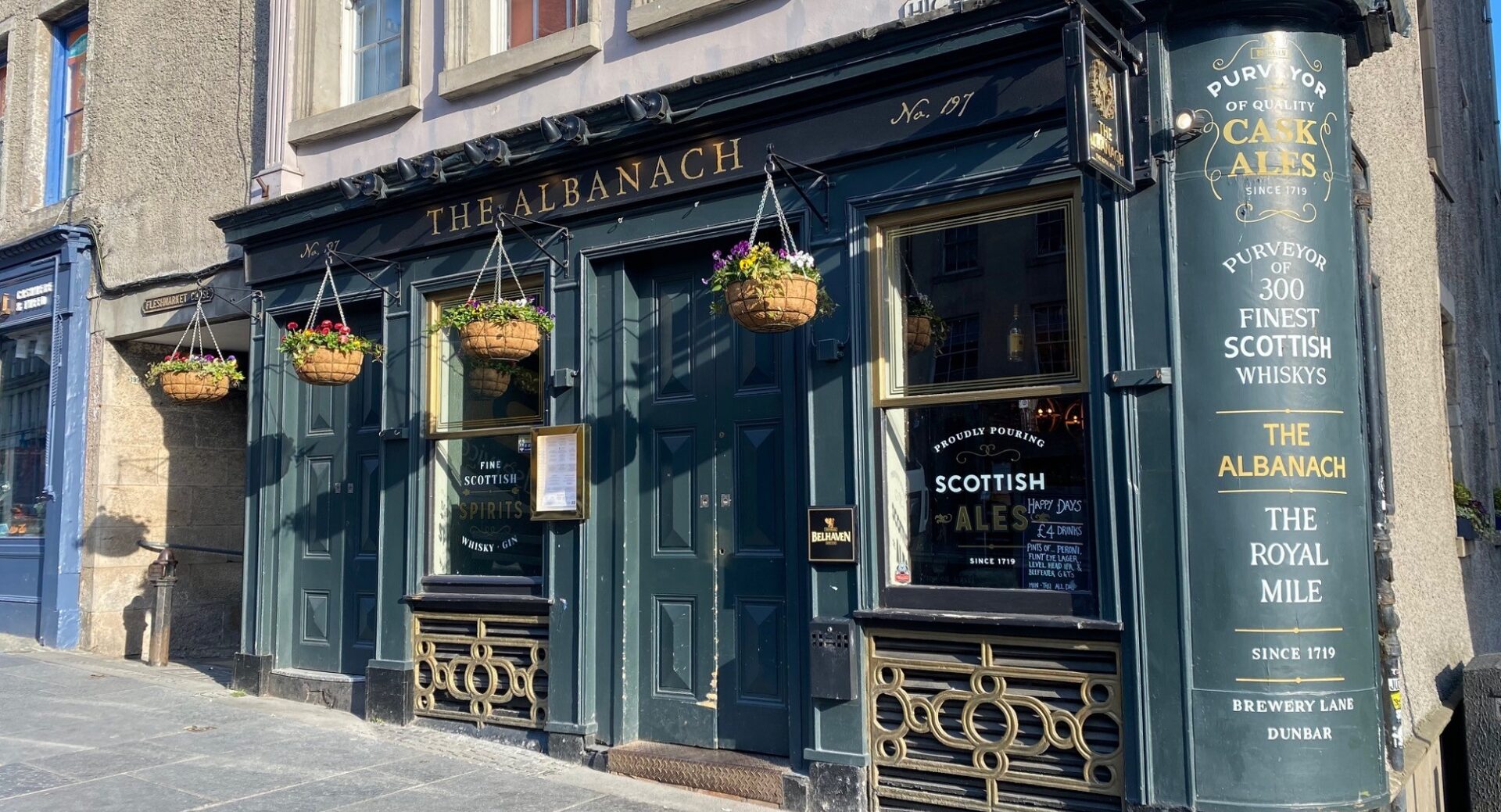The photograph captures a picturesque storefront named "The Albinac," nestled within a large, multi-story townhouse painted a rich shade of green with dark blue hues. The storefront is designed in a classic 19th-century style, featuring two double-door entrances made of wood, adorned with matching dark blue paint. On either side of the doors are rectangular windows framed in gold, with prominent signage running across the top of the storefront, highlighted by multiple black spotlights.

The signboard at the top is inscribed with the name "The Albinac" in elegant, gold serif-style font, along with the number "No. 197." Below the main signage, the storefront’s rounded corner presents further details in gold text, reading: "Purveyor of Quality Cask Ales Since 1719," and "Purveyor of 300 Finest Scottish Whiskeys - The Albinac - The Royal Mile Since 1719 - Brewery Lane, Dunbar." Additional text on the windows proudly declares: "Proudly Pouring Scottish Ales Since 1719." The scene is completed with potted plants hanging around the top portion of the storefront, adding a touch of greenery to its charming facade. The lower part of the image shows a portion of the sidewalk, emphasizing the street-level perspective typical of a bustling urban setting.